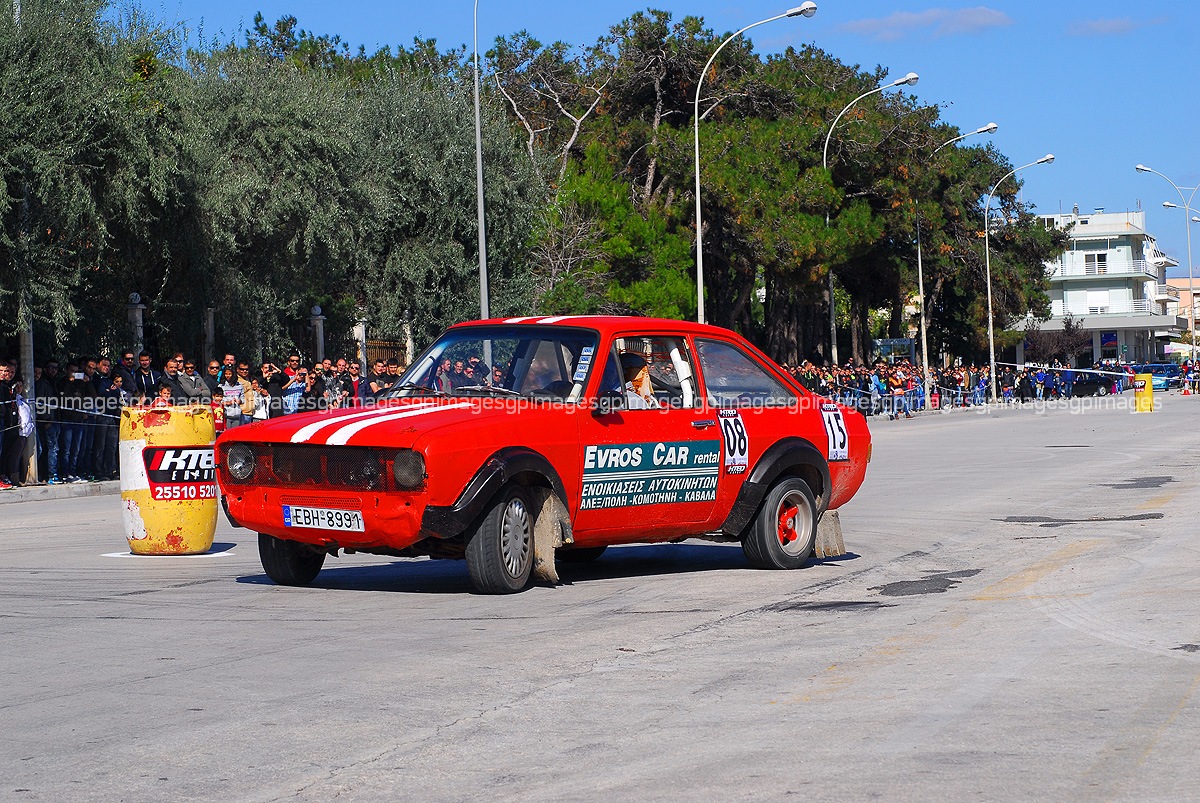The image depicts an old muscle car in a vibrant red color with two white racing stripes running down its center. The car, marked with the number plate "EBH 8991," is positioned on a gray pavement, likely in the midst of a car race or a car show. The vehicle has distinctive white squares on its side bearing the numbers "08" and "15," and the words "Evros Car Rental" are prominently displayed on the door. A yellow barrel with the letters "IKTE" and some smaller, unreadable text is situated to the left of the car. Additional details include a red bar with somewhat illegible numbers, among which "25510" and "63" are discernible. The driver, a blonde-haired individual, sits in a cockpit-like area of the car, which features a rectangular front and a front license plate reading "EBH 8991." In the background, a crowd of spectators lines the roadside, flanked by street lights and buildings. Dense, green trees are also visible under a clear blue sky, completing the scene.